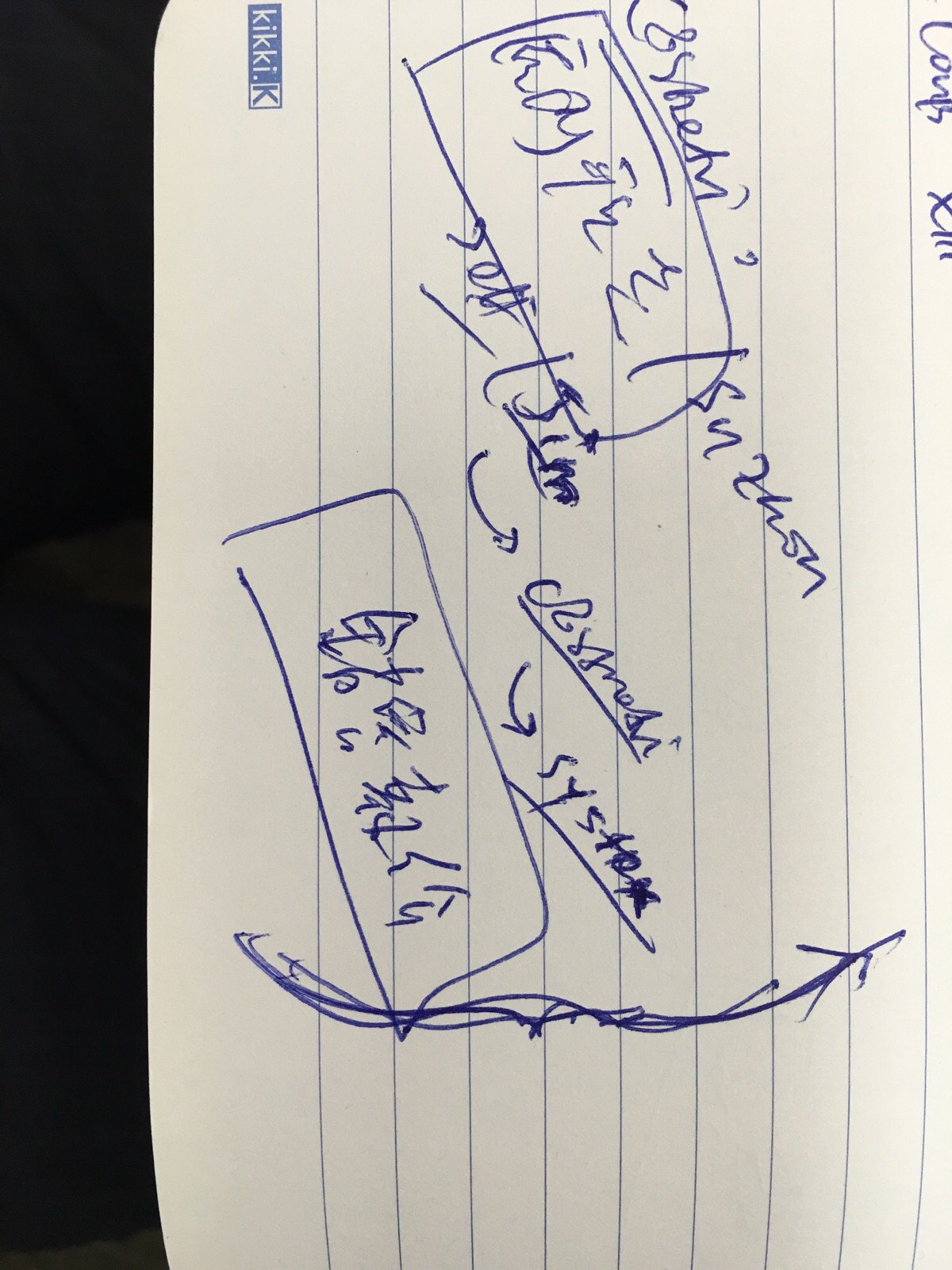The photograph captures a white piece of paper positioned at a slight angle. The paper is bordered in black on one side and features blue lines, commonly seen in notepads. Along the left margin, the letters "KI KK I K" are prominently displayed in capital letters. At the very top line, the characters "L O O P S X I I I" are written out. Below this, the word "SYZHON" appears, slanted across the paper. 

On the left side, there's a rough drawing of a square, and next to it, a rectangular shape contains several words, albeit in somewhat poor handwriting. These words seem to spell out "KZOY," followed by another "Y" with a line over it and then "EE." Beneath this rectangle, the word "self" is underlined, followed by a slash, and then the underlined word "Jim" (spelled "J I M"). An arrow points from these to the word "CRSNODI," which is also underlined. Another small arrow points from "CRSNODI" to the word "system," which is underlined as well. 

To the right of these annotations is a long, slightly curved line that appears to have been retraced multiple times. At the bottom of the page is another rectangular shape featuring more scribbles, adding to the chaotic and somewhat haphazard appearance of the document.